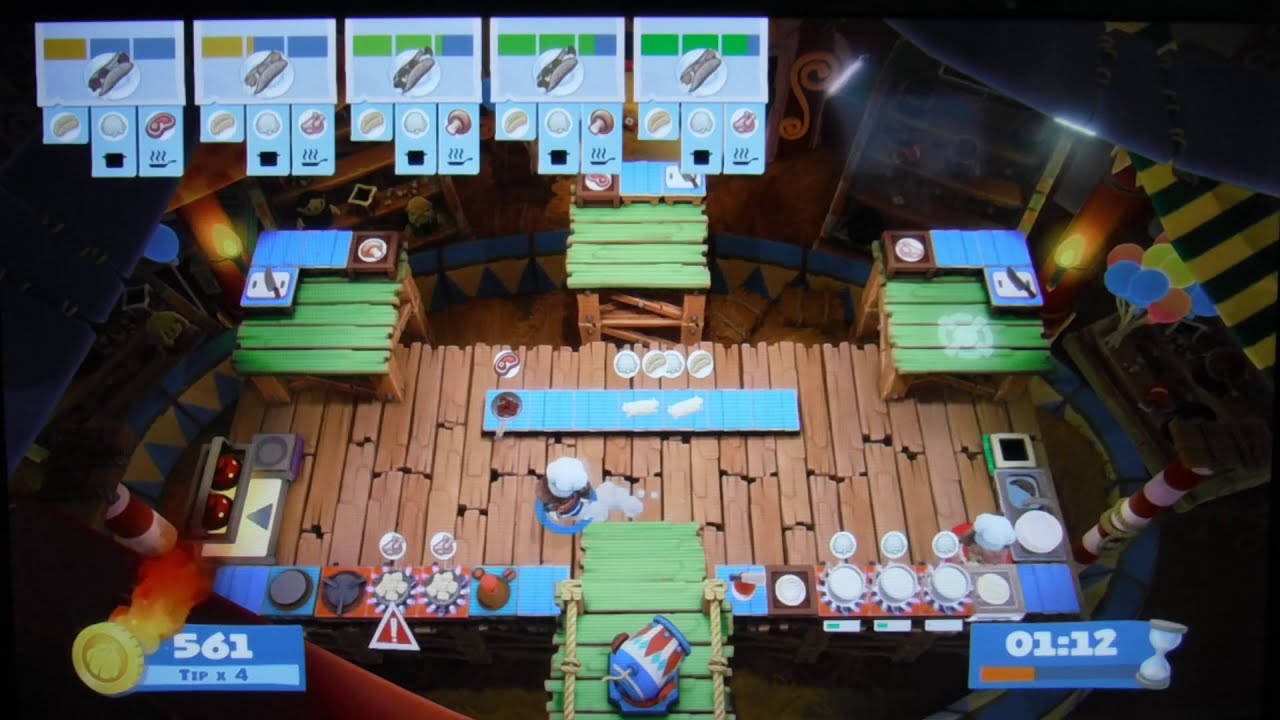The image is a detailed screenshot of a mobile or tablet cooking arcade game with a top-down view. The central feature is a wooden table, composed of interconnected wooden planks, with a green area in the middle and three green stand-up tables on the left, middle, and right sides, indicating food placement zones. To the bottom left, a blue rectangle displays the text "561 Tip x 4" with an icon of a coin engulfed in orange flames. The bottom right shows another blue rectangle featuring a timer with orange status, set at 1 minute and 12 seconds.

In the middle of the screen, there's a green wooden bridge with a cannon pointing in various directions, flanked by colorful balloons, and a candy cane-striped pole indicating an enclosed segment of the restaurant. The gameplay involves managing different cooking tasks with cartoonish characters. One character is moving from right to left toward stovetops that are at risk of boiling over, denoted by a red triangle with an exclamation mark. Another character is at the bottom right, tending to three boiling pots of rice. 

The top left of the screen shows five objects with status bars in orange, blue, and green, representing different food items like hot dogs, steaks, eggs, mushrooms, and a turkey. On conveyor belts throughout the scene, there are plates and pots containing these food items.

In summary, the image portrays a vibrant, busy cooking game environment with various status indicators, cooking stations, and characters actively engaged in preventing kitchen mishaps while managing food orders.